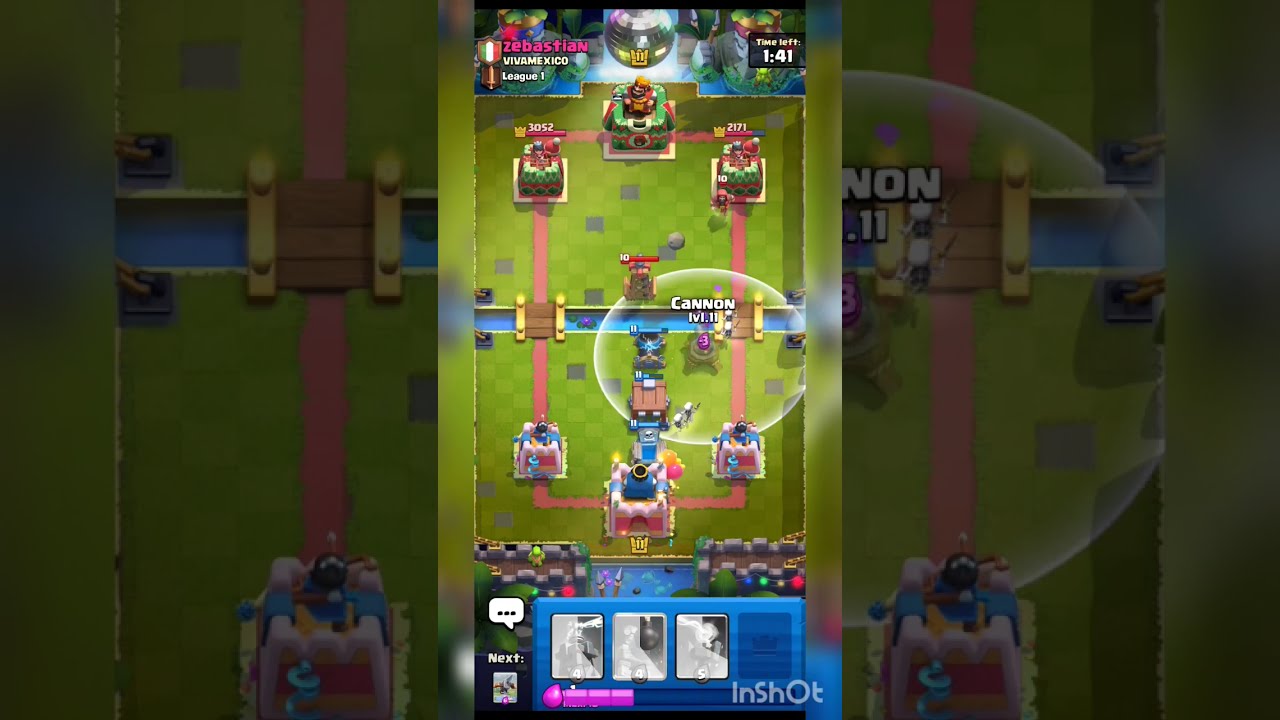This screenshot captures an intense moment from a mobile video game, featuring a dynamic playing field framed by darker, enlarged sections of the game itself. Dominating the top left corner is the name "Sebastian" in vibrant pink font, accompanied by a green, yellow, and red shield to the right, possibly indicating a national affiliation. Below "Sebastian" is white lettering, suggesting it could be a slogan or additional identifier. Adjacent to this is a glass disco ball, adding a whimsical element to the scene, followed by an indiscernible image. To the right, a black box prominently displays a game timer reading "1 minute, 41 seconds."

Central to the image is the rectangular playing field, divided into vibrant blues, pinks, and greens, with mechanical players—pinkish-reddish at the top and blue at the bottom—engaged in battle. The battlefield is punctuated by a blue area stretching horizontally through the center and a small cannon positioned strategically within the fray.

The gameplay field is structured with three smaller squares at both the top and the bottom, indicative of player positions or objectives. Below this, another blue area features four additional squares, annotated with "in shot" to the right and "next" to the left. Above "next" floats a speech bubble, suggesting in-game communication or alerts.

At the very bottom, a logo reading "inShot" (small i, small n, capital S, small h, capital O, small t) potentially identifies either the game or its creator. Lastly, a partially filled pink ticker runs along the bottom, likely reflecting game progress or loading status, completing this richly detailed snapshot of a mobile gaming experience.